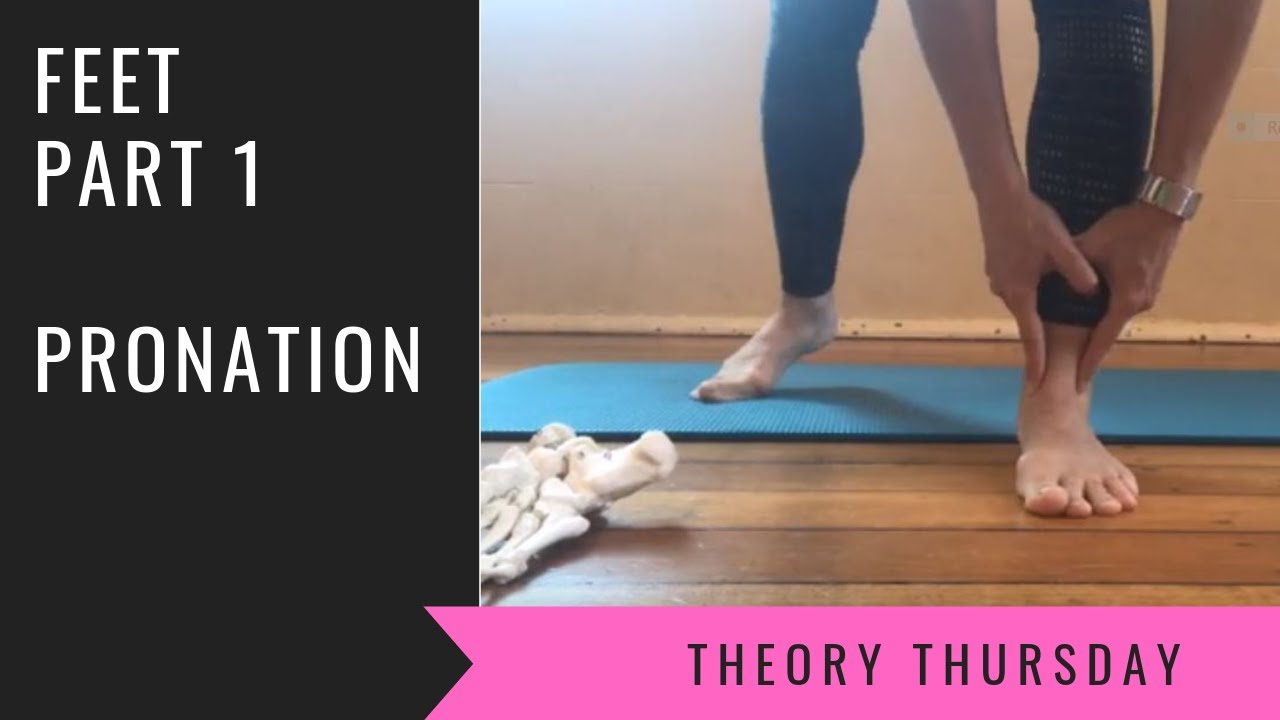The image is a detailed health advisory guide focusing on feet, specifically on the topic of pronation. The slide is divided into distinct sections: on the left, a black box with white text prominently displays the title "Feet, Part One: Pronation." In the bottom center, a hot pink banner with black letters reads "Theory Thursday." The right two-thirds of the slide features an illustration showing a pair of legs from the knees down. The person, likely a woman in yoga pants, is standing with one foot forward on a wooden floor and the other foot back on a blue yoga mat. She is bending over, using both index fingers to touch her left ankle, seemingly checking for pain or lumps. Beside her, closer to the middle of the slide, is a model of foot bones, suggesting an educational presentation on flat feet or a related condition.